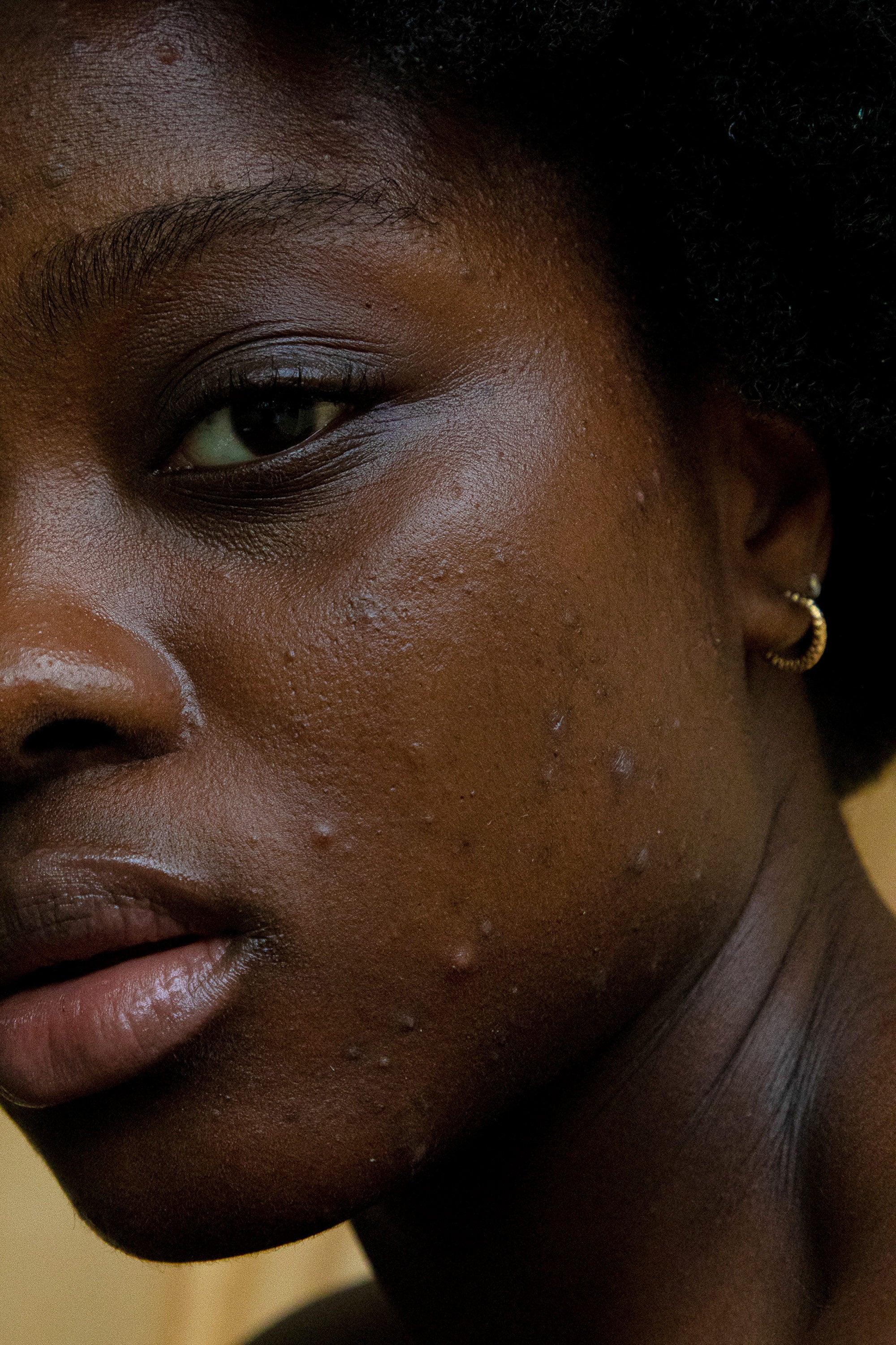This photograph captures the side profile of a young, dark-skinned African-American woman in her 20s. The image focuses on her left side, showcasing her left eye, half of her nose, and her lips, which are slightly parted and have a slight pink hue. Her black hair is styled up, not down to her shoulders, allowing a clear view of her facial features, including her nicely shaped eyebrows and expressive eyes. She exhibits a neutral expression as she gazes at the camera. Her skin, while possessing some acne and scars particularly on her left cheek and forehead, appears healthy. Her ear is adorned with a small gold hoop earring and an additional diamond stud. The background is a vibrant yellow, and the lower part of the image reveals her neck, implying she has no shirt on, with the focus remaining from her neck upwards.